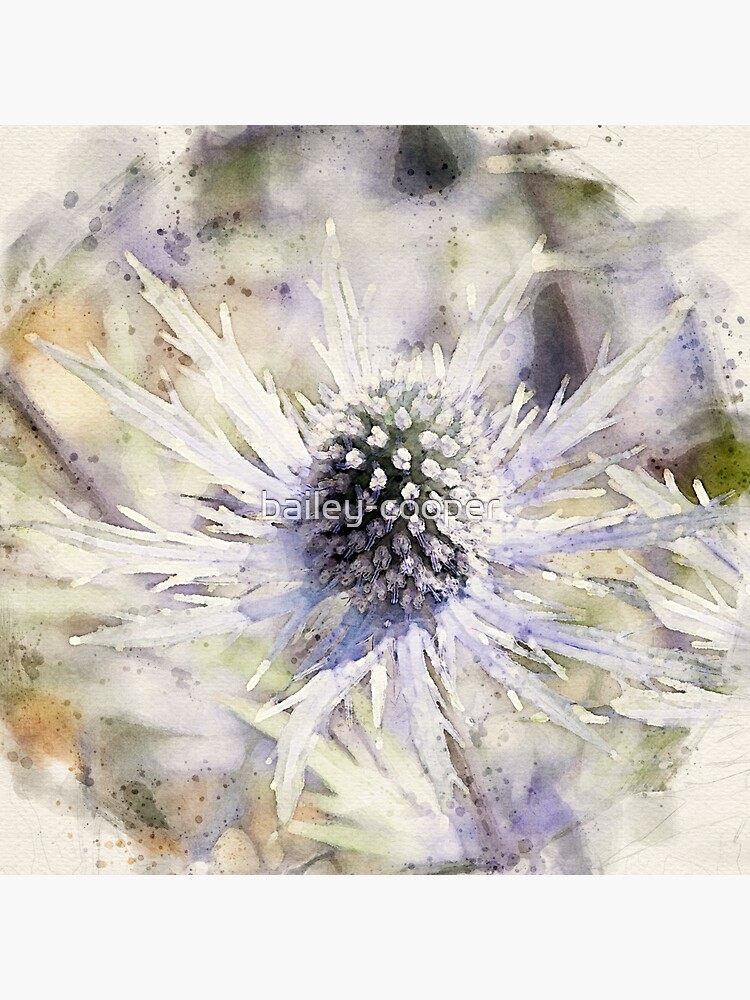This image depicts an artist's watercolor drawing of an extreme close-up view of a flower's interior. The focal point of the image is a central flower bud, resembling a pine cone, adorned with muted white and purple tips, which radiates a combination of greenish, grayish, and purplish hues. Surrounding this center are serrated-style petals, primarily white with a faint purple hue, extending outward in all directions. The background features an artful blend of purples, greens, yellows, beiges, and oranges, with a blurring and blending effect punctuated by speckles of more intense colors. A translucent white watermark with the name "Bailey Cooper" is centered within this intricate composition.